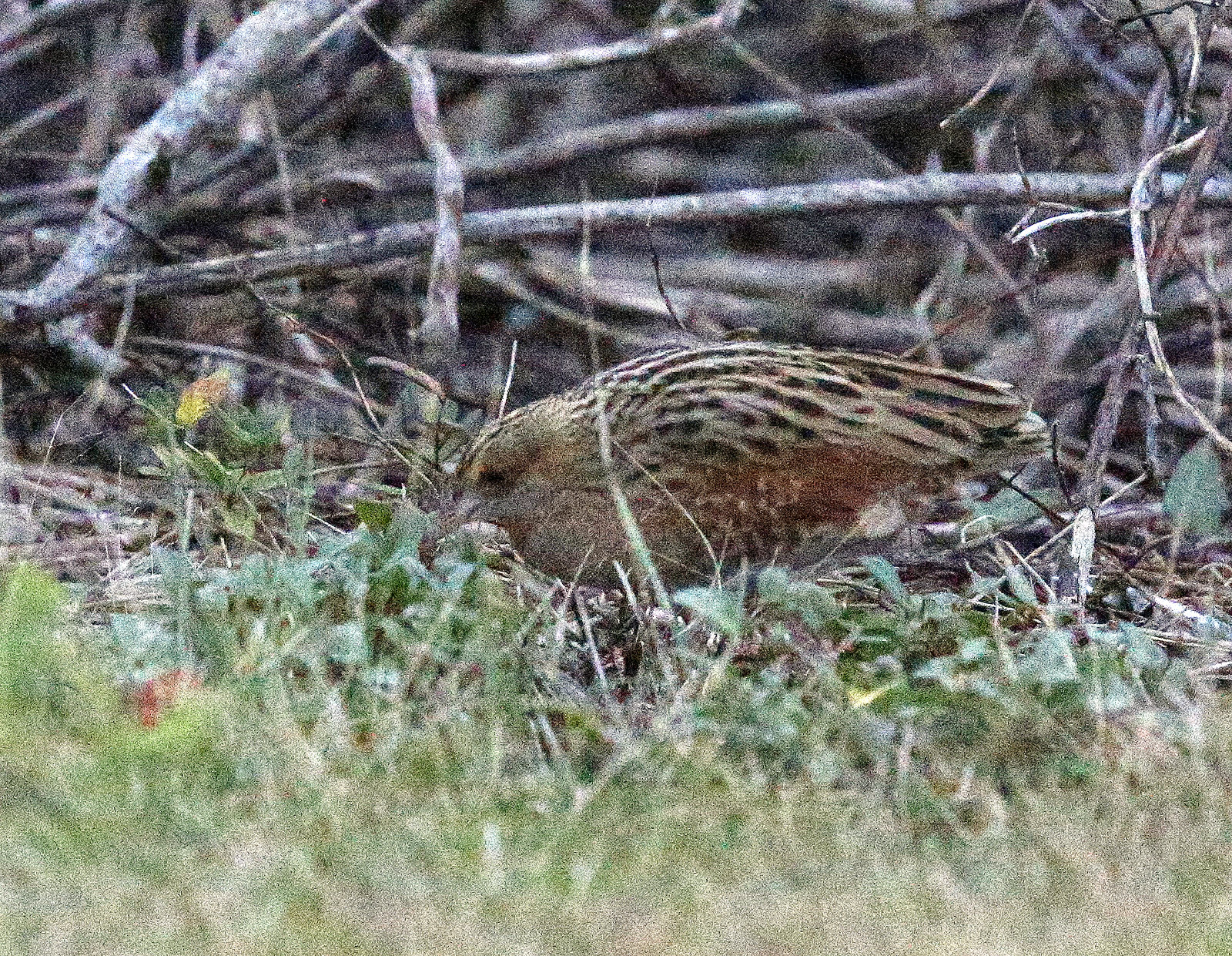The photograph captures a small bird in a natural setting, resting on the ground amidst a foreground of grass that appears washed out in white but transitions to a greener hue near the bird. The bird, seen in profile from right to left, has a brownish plumage with a lighter belly and neck, and a darker back. Its wings exhibit speckled black and white patterns, while its back end has a reddish tint. The bird's small beak is mostly obscured by the grass as it appears to peck at something on the ground. Surrounding the bird in the background is a thicket of branches and interwoven twigs, featuring a distorted greenish-brown color, creating a somewhat grainy and dimly lit atmosphere. The scene gives an impression of a possible nesting area, although it seems rather large for a typical bird nest.